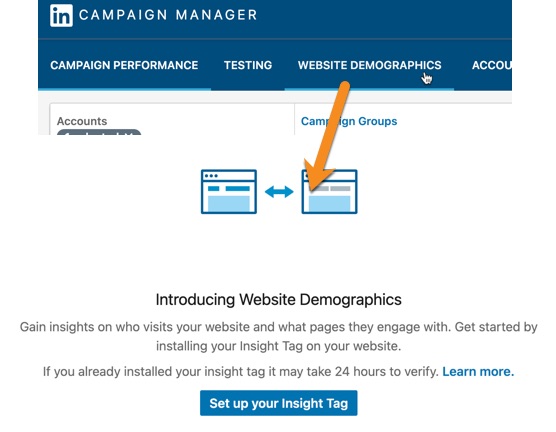The image features a dark blue border along the top, prominently displaying the LinkedIn logo in the top left corner. To the right of the logo, in bold white capital letters, are the words "Campaign Manager." Below that, several options are listed in smaller white text: "Campaign Performance," "Test Website Demographics," and "Account." A white-gloved hand points specifically to the option labeled "Demographics." 

Underneath this section, there is a bordered box labeled "Accounts," followed by another labeled "Campaign Groups." Between these boxes, two file icons are illustrated, depicting the sharing of files, with an orange arrow pointing to the file on the right. 

Further down, the image introduces a feature called "Website Demographics," providing a detailed explanation:
"Introducing Website Demographics, gain insights on who visits your website and what pages they engage with. Get started by installing your Insight Tag on your website. If you have already installed your Insight Tag, it may take 24 hours to verify." 

There is a "Learn More" hyperlink for additional information, and a prominent blue box that encourages users to "Set Up Your Insight Tag."